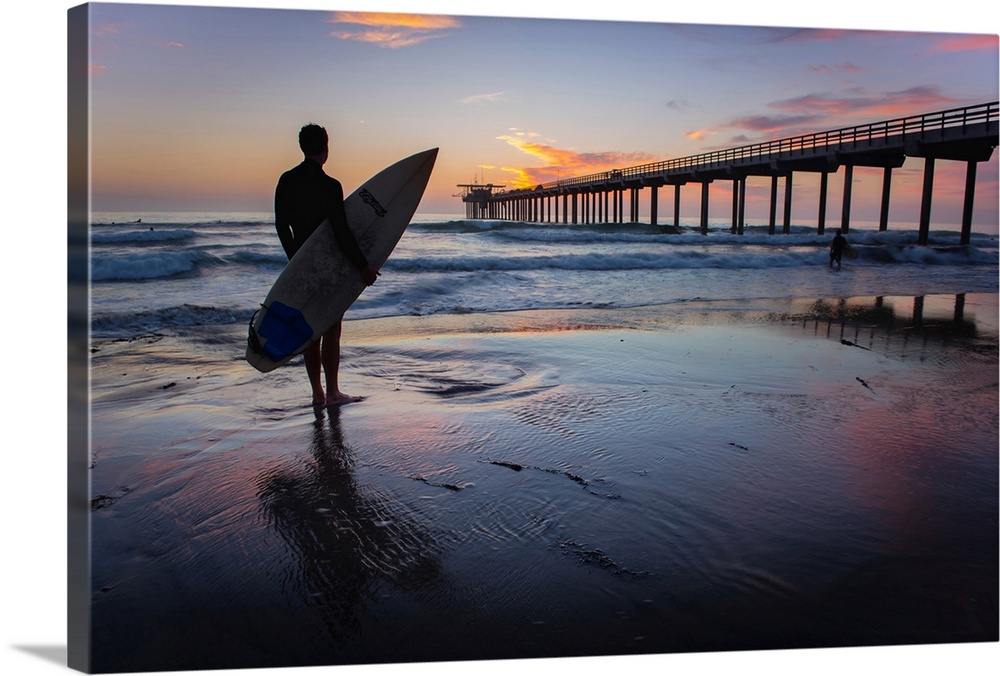A stunning beach scene at sunset unfolds in this image. The sky is an exquisite blend of light blue transitioning to hues of gold, orange, pink, and purple as the sun begins its descent towards the horizon. Wisps of golden-tinted clouds add depth and warmth to the scenery. Below, the calm blue water mirrors the sky's vibrant colors, creating a serene and reflective surface. The wet sand at the shoreline glistens from the recent touch of the waves. A surfer, accompanied by a young man, stands poised with a surfboard under his arm, ready to embrace the ocean's call. To the right, a towering bridge elegantly spans across the water, adding a dramatic architectural element to the scene. In the distance, a large ship sails by, while other beachgoers can be seen enjoying the water, contributing to the dynamic and lively atmosphere of this picturesque setting.